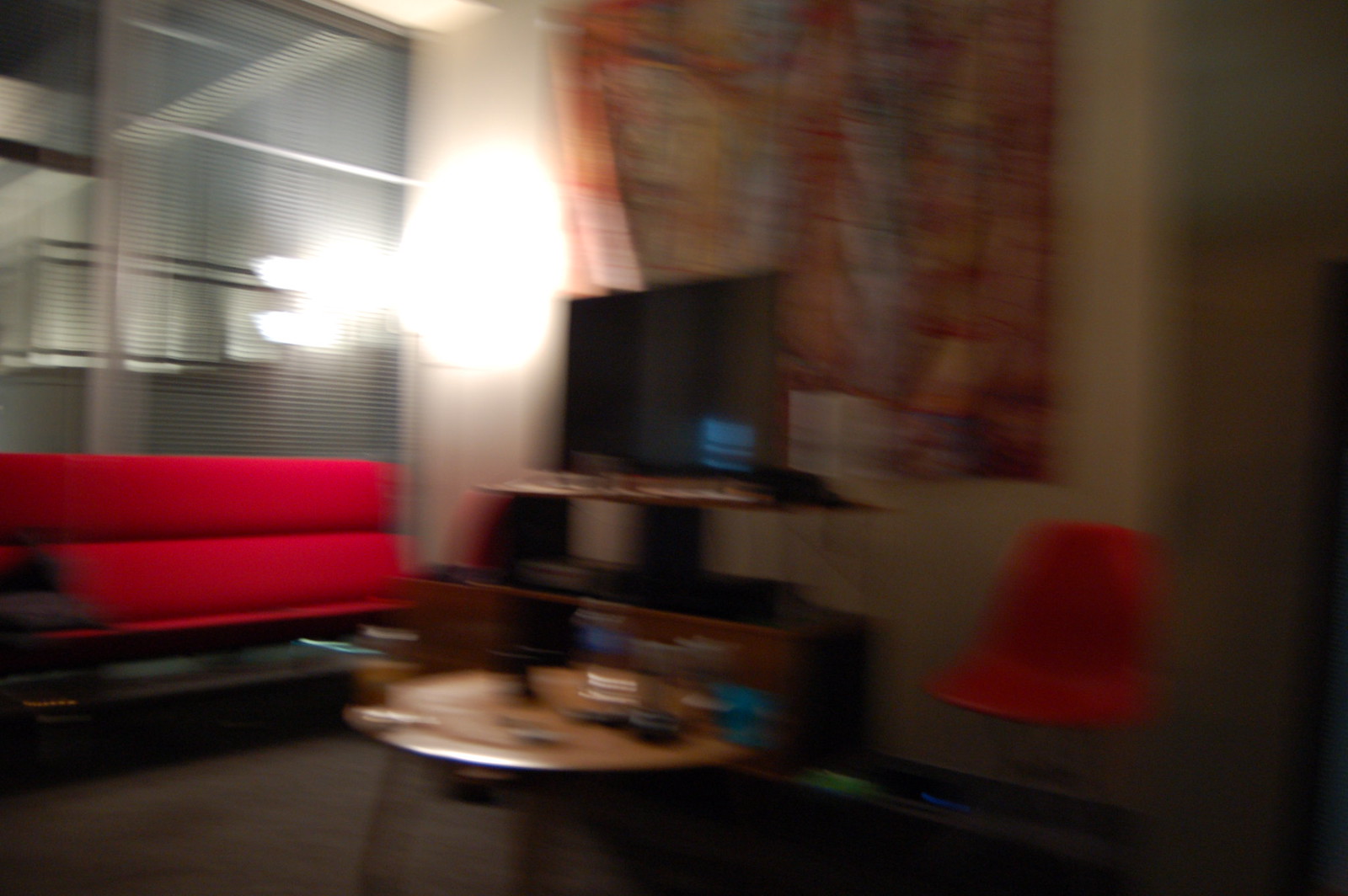A slightly blurry image captures the interior of a cozy apartment living room. The walls are painted white, setting a clean and neutral backdrop. Dominating one section of the wall is a large hanging fabric with an intricate orangish-blue pattern, adding a touch of color and texture.

At the center is a wooden TV stand supporting a medium-sized black flat-screen TV. To the right of the stand, a red plastic chair without arms adds a pop of color. On the left side, large glass windows allow natural light to flood the room, complemented by a bright, modern lamp positioned next to them, enhancing the room's ambiance.

A stylish red couch sits prominently, offering a place to relax. The floor is covered with a grayish carpet that grounds the room with a soft, inviting feel. At the center of the carpet, a round wooden coffee table holds an assortment of miscellaneous items, among which certain objects remain unidentifiable, adding an element of lived-in comfort.